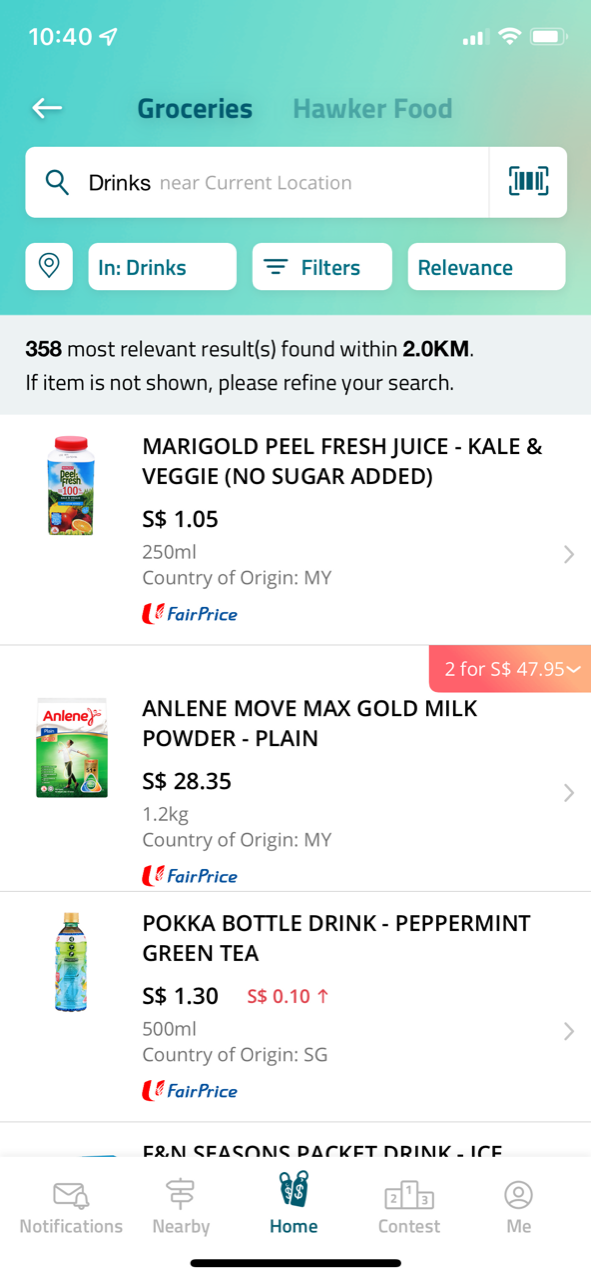This is a detailed screenshot taken from a phone, displaying a search results page for groceries within a specific app. 

In the upper left-hand corner, the time is displayed as 10:40 AM, and beside it, there's a send arrow icon. On the right-hand side, a nearly full signal strength icon is visible, followed by a fully filled Wi-Fi icon, and then an almost fully charged battery icon.

Below the status bar, on the left-hand side, there is a back arrow pointing to the left. Next to the arrow, "Groceries" is prominently bolded in black, followed by "Hawker Food." Directly below this, there is a search bar with a magnifying glass icon and the text "Drinks." Beside the search bar, in light gray text, it says "Near Current Location." At the far right end of this bar, there's a barcode scanning icon.

Beneath the search bar, a location pin icon is followed by "In Drinks, Filters, Relevance." Below this line, a gray banner states "358 most relevant results found within 2 KM. If item is not shown, please refine your search."

Following the banner, three products are listed:

1. Marigold Peel Fresh Juice, Kale and Veggie, No Sugar Added – priced at $1.05, labeled with "Fair Price."
2. Anlene MoveMax Gold Milk Powder, Plain – priced at $28.35, with a special offer of 2 for $47.95, also labeled "Fair Price."
3. Pokka Bottle Drink, Peppermint Green Tea – priced at $1.30, also labeled "Fair Price."

At the bottom of the screen, there are some icons, presumably for additional actions or navigation.